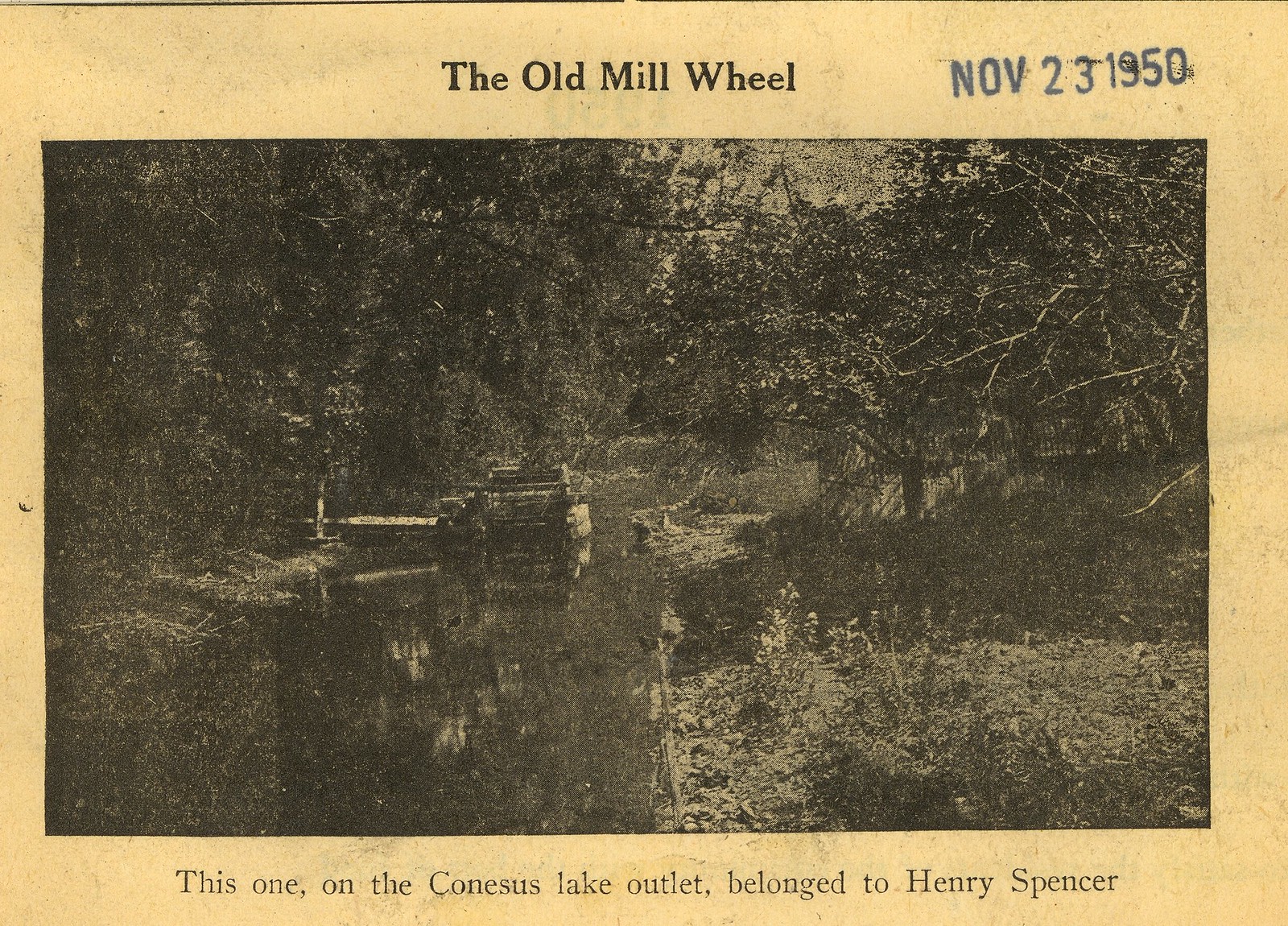The image is a significantly aged and yellowed black-and-white photograph from November 23, 1950. Titled "The Old Mill Wheel" at the top, the photograph portrays a water area identified as the Conesus Lake outlet, once belonging to Henry Spencer. The image quality is poor and blurry, making the exact details challenging to discern. However, it appears to capture a mill wheel in a river or stream, flanked by abundant trees and grass. The text at the bottom confirms its location and ownership, providing a historical context to the scene.